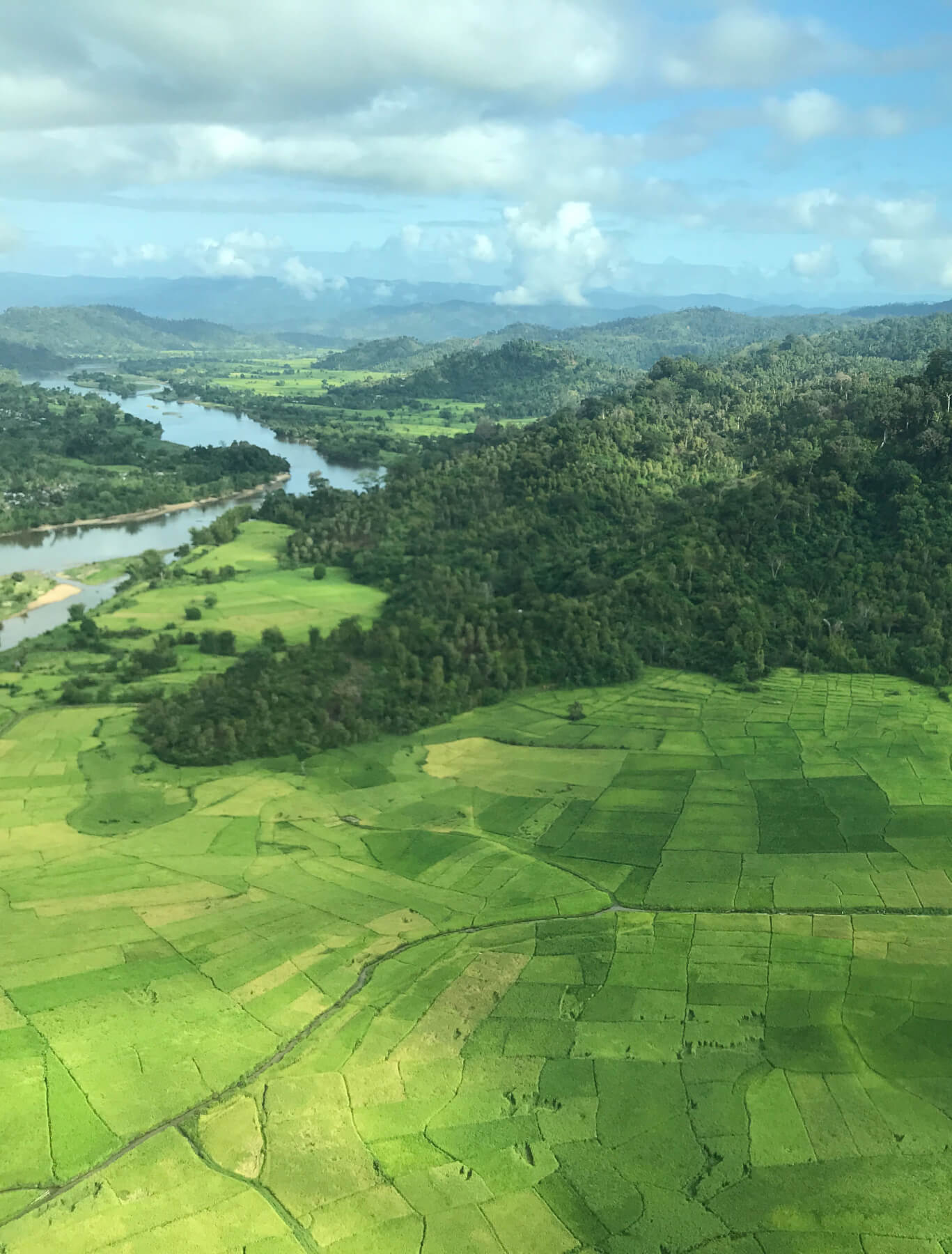The aerial photograph captures a vast and picturesque landscape divided into distinct layers of natural beauty and human cultivation. The sky, a serene light blue, is peppered with various large, fluffy white clouds. In the distance, heavily hilly terrain is blanketed with a dense, lush tree line, transitioning to mountainous regions that appear blue further back. A river winds gracefully through the valleys, entering from the center left and continuing off into the horizon.

In the foreground, the land is dominated by multiple cultivated fields, each plot with vibrant green crops varying in shades from light to dark green, intersected by noticeable pathways and smaller roads. A primary road runs diagonally from the bottom left corner to the bottom right, with several smaller branches spreading out from it, seamlessly weaving through the expansive farmland. These fields are meticulously sectioned and flat, hinting at careful agricultural use. The fusion of hilly woodlands and structured farmlands creates a stunning contrast, encapsulating the beauty of both natural and man-made landscapes.